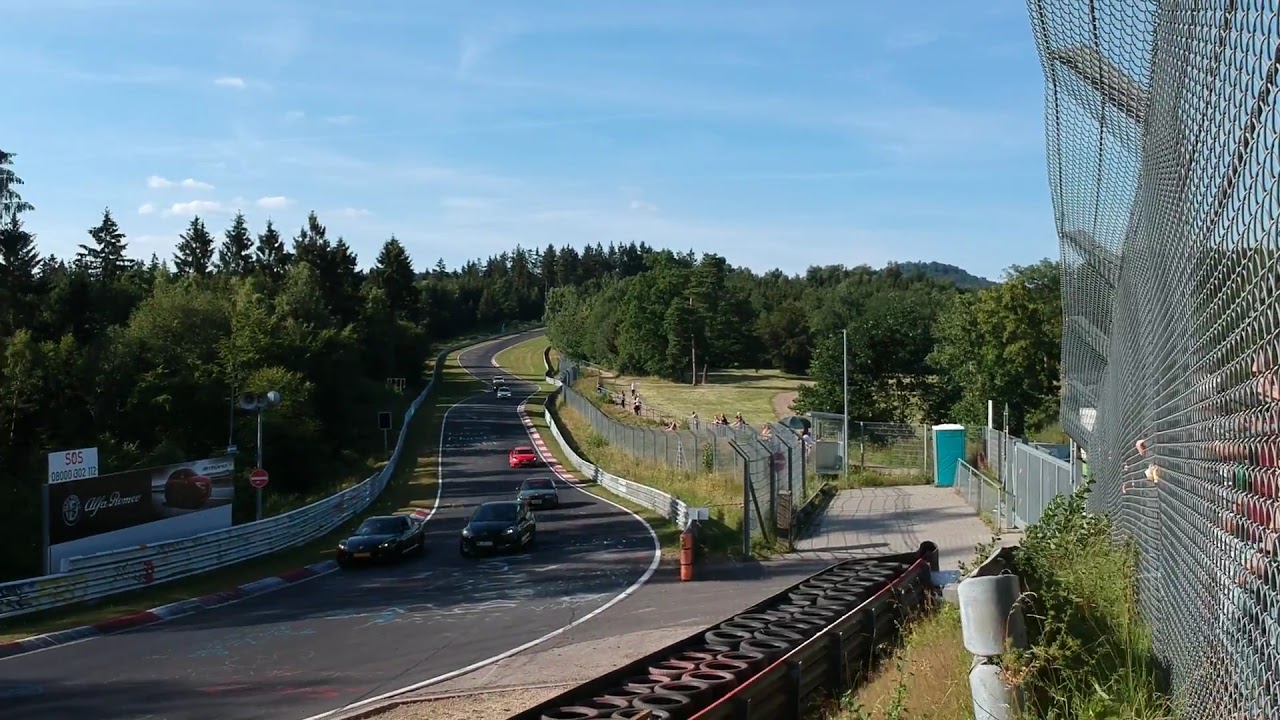The image captures a vibrant scene of a winding, one-way asphalt street that appears to be part of a racetrack descending a steep hill. The street, occupied by six cars — two black cars at the forefront, followed by a dark green car, a red car, and some indistinguishable cars in the distance — is bordered by a series of barriers. The barriers include stacked tires with metal plates on either side and high chain-link fences. To the right side of the image stands a mint green port-a-potty with a white roof. 

Spectators are gathered behind the fences, appearing to be around a dozen in number, scattered across various sections, likely engrossed in the racing action. In addition to the barriers, a sign reading "Alpha Premier 505" is visible on the left side of the image. Both sides of the track are lined with dense vegetation, featuring an abundance of green trees and patches of brush, creating a picturesque, leafy backdrop. The sky above is partly cloudy with mostly blue patches, framing the dynamic scene below.